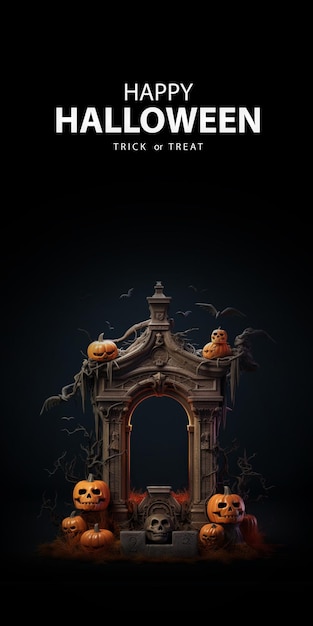The image showcases a dark and eerie Halloween-themed scene. Dominating the frame is a black background that adds an ominous atmosphere. At the top of the image, a sign prominently reads "Happy Halloween" with "Happy" in slightly smaller letters and "Halloween" larger for emphasis. Below this, in even smaller letters, "trick-or-treat" is inscribed, reinforcing the Halloween theme.

At the bottom of the image, there's a collection of intricately carved jack-o'-lanterns arranged around a high-arched gravestone-like structure, adding to the spooky ambiance. On the left side, three pumpkins with sinister faces are grouped together while on the right side, two more pumpkins are placed. In the middle of this arrangement, there's a particularly unnerving figure resembling either a skull or a creepy clown face, heightening the unsettling mood.

Further up, resting atop the arched structure, are two more jack-o'-lanterns with strange, exaggerated expressions. Additionally, there are two more pumpkins on the left side, one featuring rosy cheeks which provide a stark contrast to the otherwise dark and grim setting. The base of the structure displays a cement-like, gray area, contributing to the gravestone appearance.

Bats are seen flying against the night sky in the background, completing this hauntingly detailed Halloween scene.